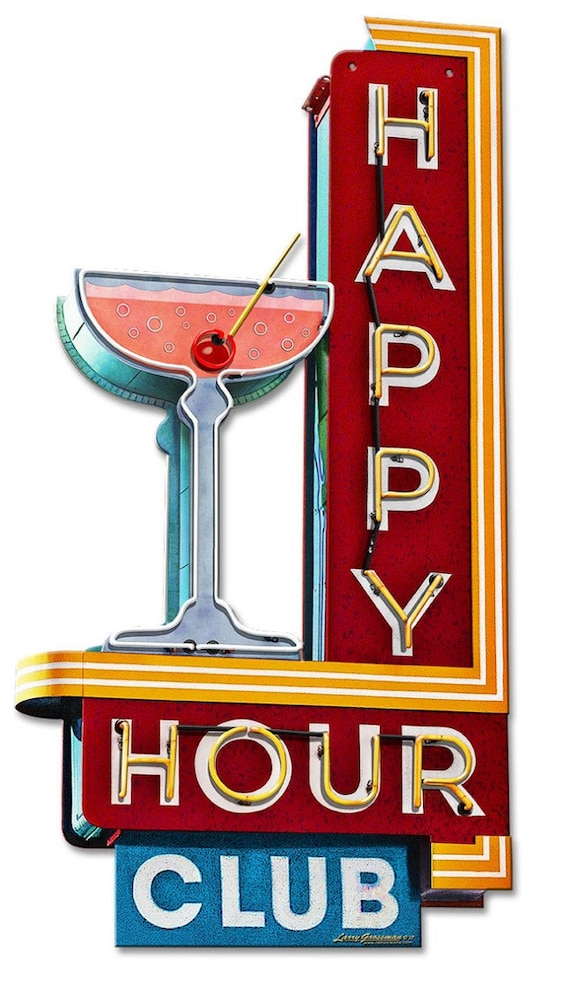The image depicts a vintage neon sign, likely from the 1950s, ideal for hanging on the side of a building or above a bar. The sign is characterized by its classic red and blue rectangular sections and prominent neon lighting. The top part of the sign features the word "Happy" in vertically aligned yellow neon tubular lettering against a red background. Adjacent to the vertical "Happy" is a martini glass filled with pink liquid, a maraschino cherry, and a green toothpick. Below this setup, a horizontal rectangle displays the word "Hour" in similar yellow neon lights on a red backdrop. Lastly, at the bottom, a blue rectangle houses the word "Club" in plain white letters without neon lighting, completing the retro design. The entire sign is set against a white background, enhancing the colorful and nostalgic aesthetic.